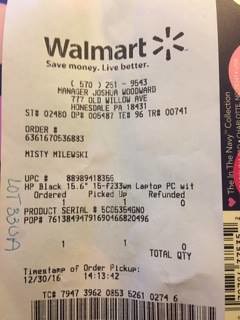In this rectangular photograph, a Walmart receipt is prominently displayed in an upright vertical position. The background of the image on the right side reveals a partial view of a barcode. Against this black backdrop, faint white text reading "The Navy Collection" is visible. The receipt details that it is from Walmart, managed by Joshua Woodward, located on Old Willow Avenue in Holmesdale, Pennsylvania. The order in question, bearing the number 6361670536883, indicates that an HP black laptop PC was ordered and subsequently picked up on December 30, 2016.